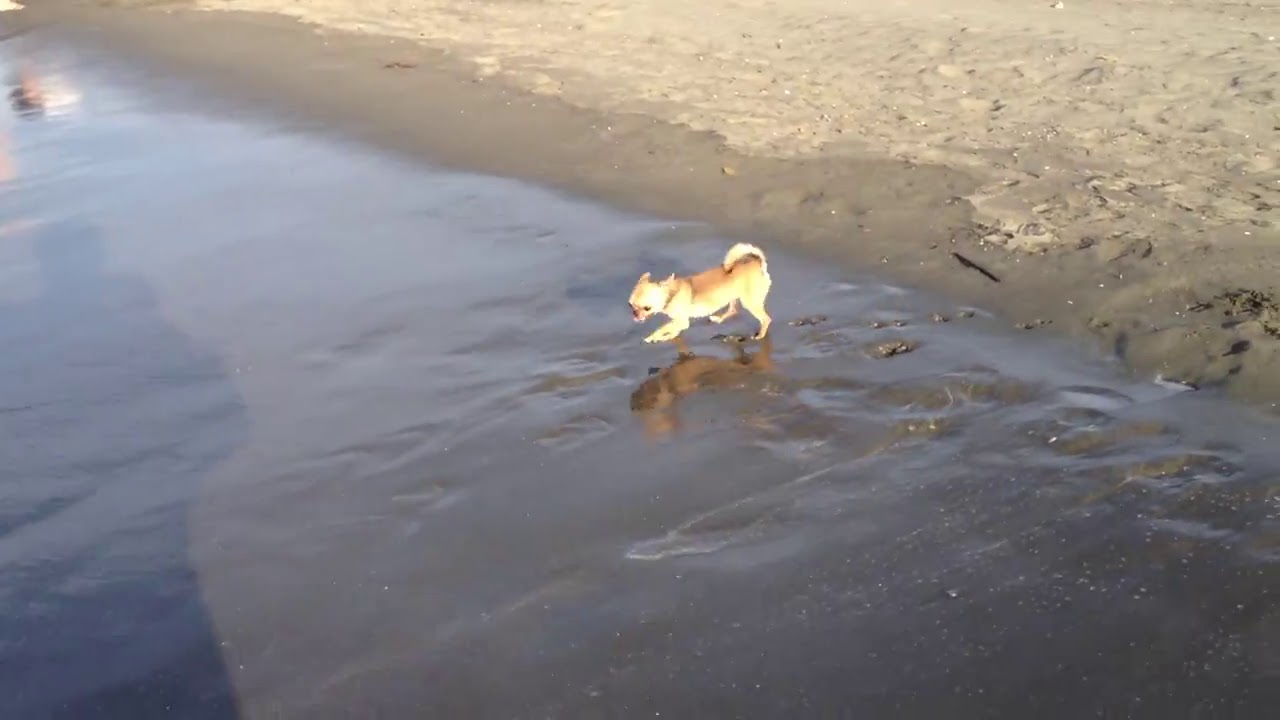A small, tan chihuahua is the focal point of this outdoor beach scene, captured in the middle of the day. The dog, with its furry tail curled upwards and tongue playfully sticking out, stands in the shallow water near the center of the image. The beach itself is muddy rather than sandy, with visible footprints trailing behind the dog. The water appears calm and clean, reflecting both the dog and a faint human silhouette in the top left corner. A prominent shadow of the person taking the picture can be seen on the bottom left, indicating they are standing at the water's edge. The color palette of the image includes earthy tones such as light brown, dark brown, and touches of yellow, alongside the muddy shoreline and the shimmering water. The overall scene also conveys a sense of tranquility and simplicity.